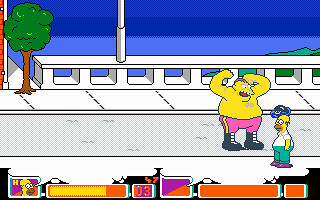This image is a screenshot from an old arcade game, specifically the Simpsons arcade game. In the bottom right-hand corner, Homer J. Simpson can be seen standing next to a large, shirtless, burly wrestler-like character wearing pink pants with a yellow stripe and tall black knee-high boots. The two characters appear to be in conflict on the side of a bridge, with Homer donning a white shirt, light green pants, and black or brown shoes. He also has a blue bag on his head and a black bowling ball beside him. The bridge features bright white sidewalks and a yellowish road, with what looks like a river or ocean indicated by bright blue water below. On the left side of the screen, there's a green tree with a brown trunk. The bottom of the screen displays a HUD with Homer's image, a health bar to the right of his face, and the number three, likely indicating his remaining lives. The health bar is reddish-yellow, and Homer's icon features an 'H' and a bordered square that's half-purple and half-red. A little flagpole is visible near the bridge as well, adding to the detailed environment of this classic video game scene.